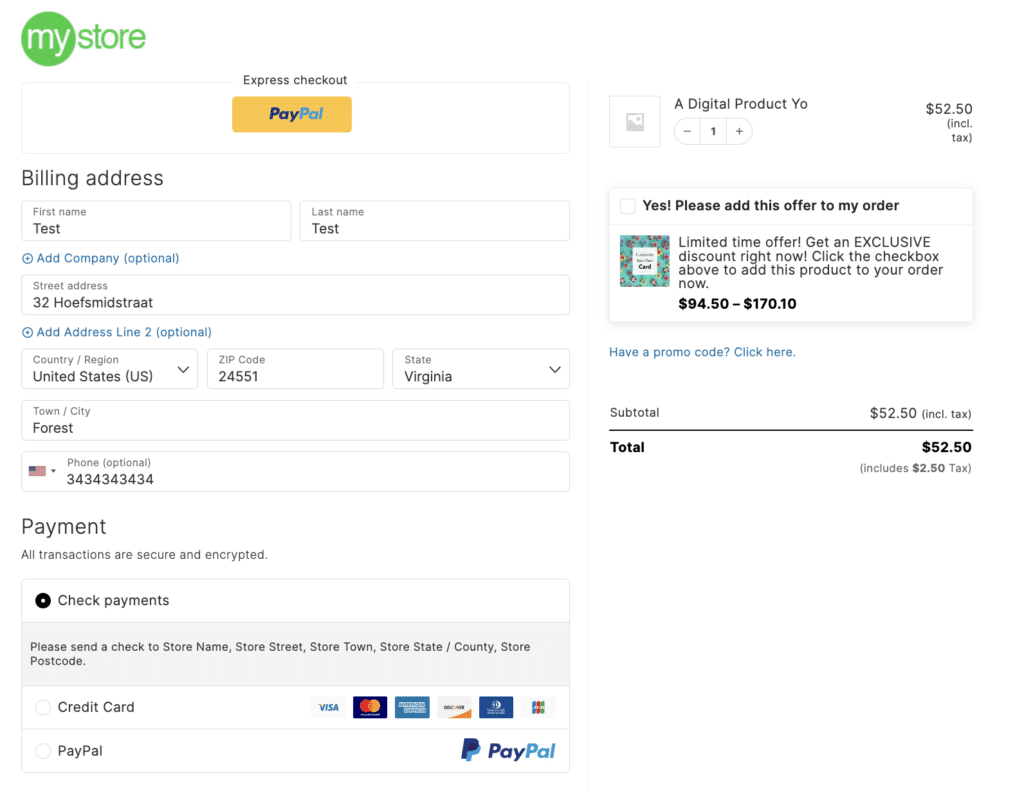The screenshot captures the express checkout page of a store named "My Store," prominently featuring its white and green icon in the upper left corner. The central part of the image includes various labeled pop-up and text boxes for user input. 

On the left, there's a detailed billing address section requiring the following details: first name, last name, street address, country, region, zip code, state, town, city, and an optional phone number. Below this section lies the payment section, which offers a choice between credit card and PayPal, indicated by respective icons and a selection circle. 

To the right, the page showcases a summary of the selected item, "Yo," with a quantity of one. The total cost for the purchase is $52.50, inclusive of tax. Beneath this summary, there is an option to add an exclusive discount to the order and a blue hyperlink for entering a promo code. The subtotal and the total amount are both prominently displayed in bold black font, $52.50.